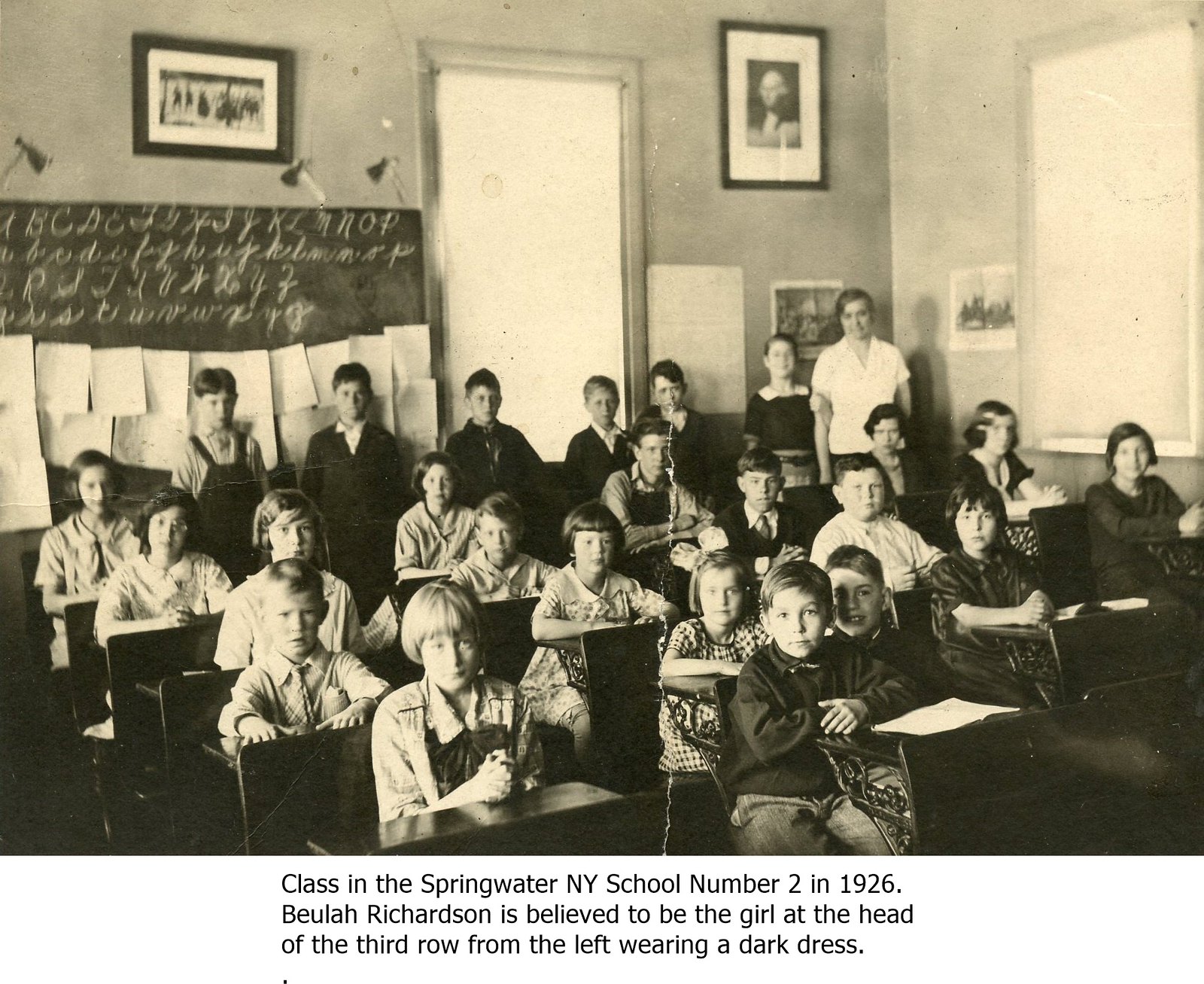This black and white photograph, dating back to 1926, captures a classroom scene at Springwater New York School Number 2. The image shows four rows of seven-year-old children, each child seated at their desk with their arms neatly placed in front of them, looking attentively toward the camera. Believed to be among the students is Beulah Richardson, who is identifiable as the girl at the head of the third row from the left, wearing a dark dress. The classroom features high ceilings, and the teacher can be seen standing in the back right corner of the room. Above her, there is a prominently displayed framed portrait of George Washington. The walls are adorned with various papers and framed photos. On the blackboard, there is handwritten cursive script displaying the alphabet in both uppercase and lowercase. Additional details such as the white banner below the photograph, which reads "Class in Springwater NY School Number 2 in 1926," further authenticate the scene's historical context.